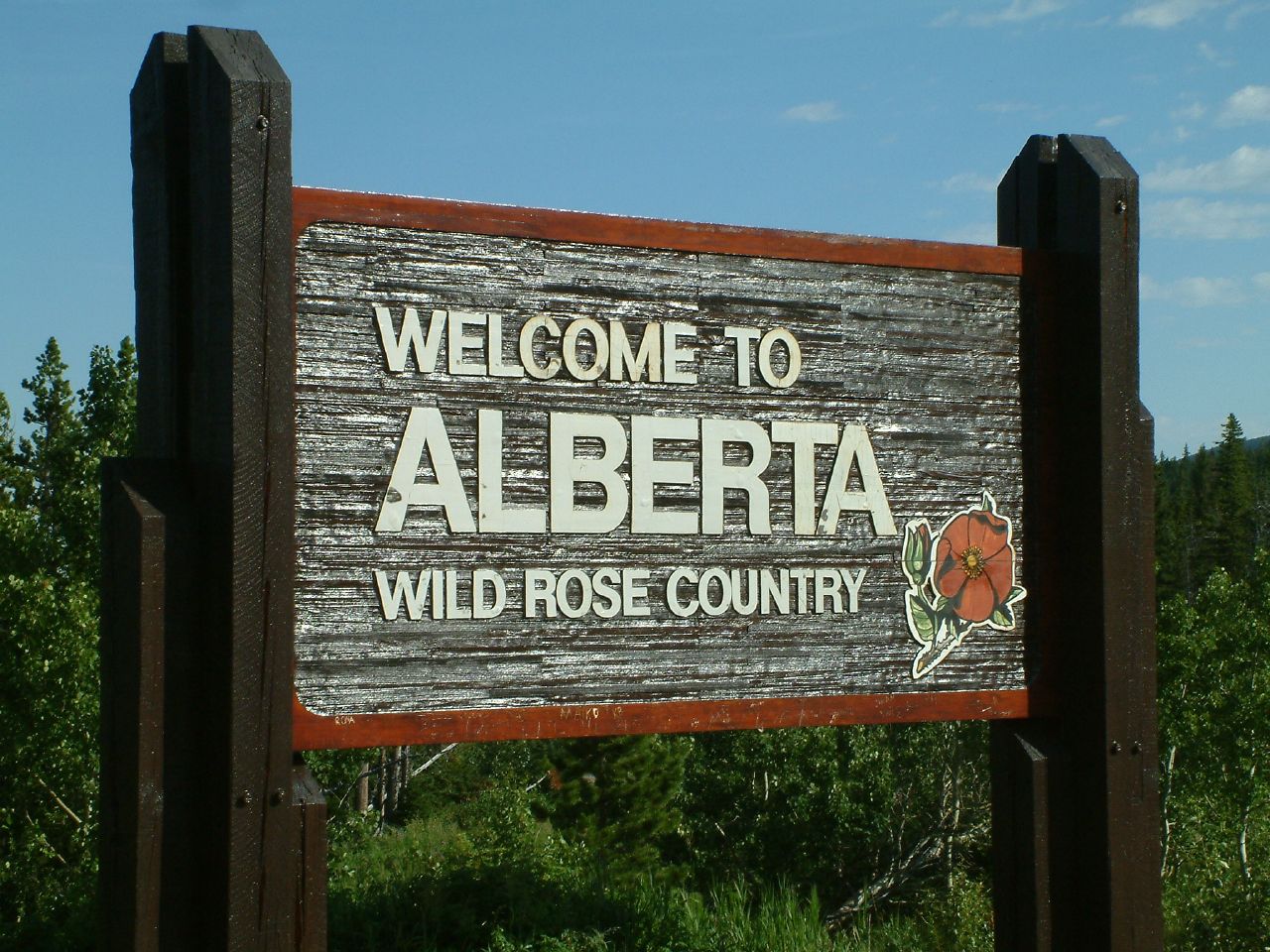The photograph depicts an outdoor scene featuring a large wooden sign held up by two brown posts. The sign itself is shiny and charcoal gray, bordered in red at the top and bottom. Prominently displayed in big white uppercase letters are the words "Welcome to Alberta," with "Alberta" being the largest. Below that, it reads "Wild Rose Country," also in white uppercase letters. In the lower right corner of the sign, there is an illustration of a red wild rose with green leaves. The sign is set in a grassy field, with an array of trees, shrubs, and bushes in the background, featuring both pine and deciduous trees. The sky above is a clear blue with some white clouds on the right side, and the sun is shining, casting noticeable shadows on the ground. In the distance on the right, a hill or mountain is visible.